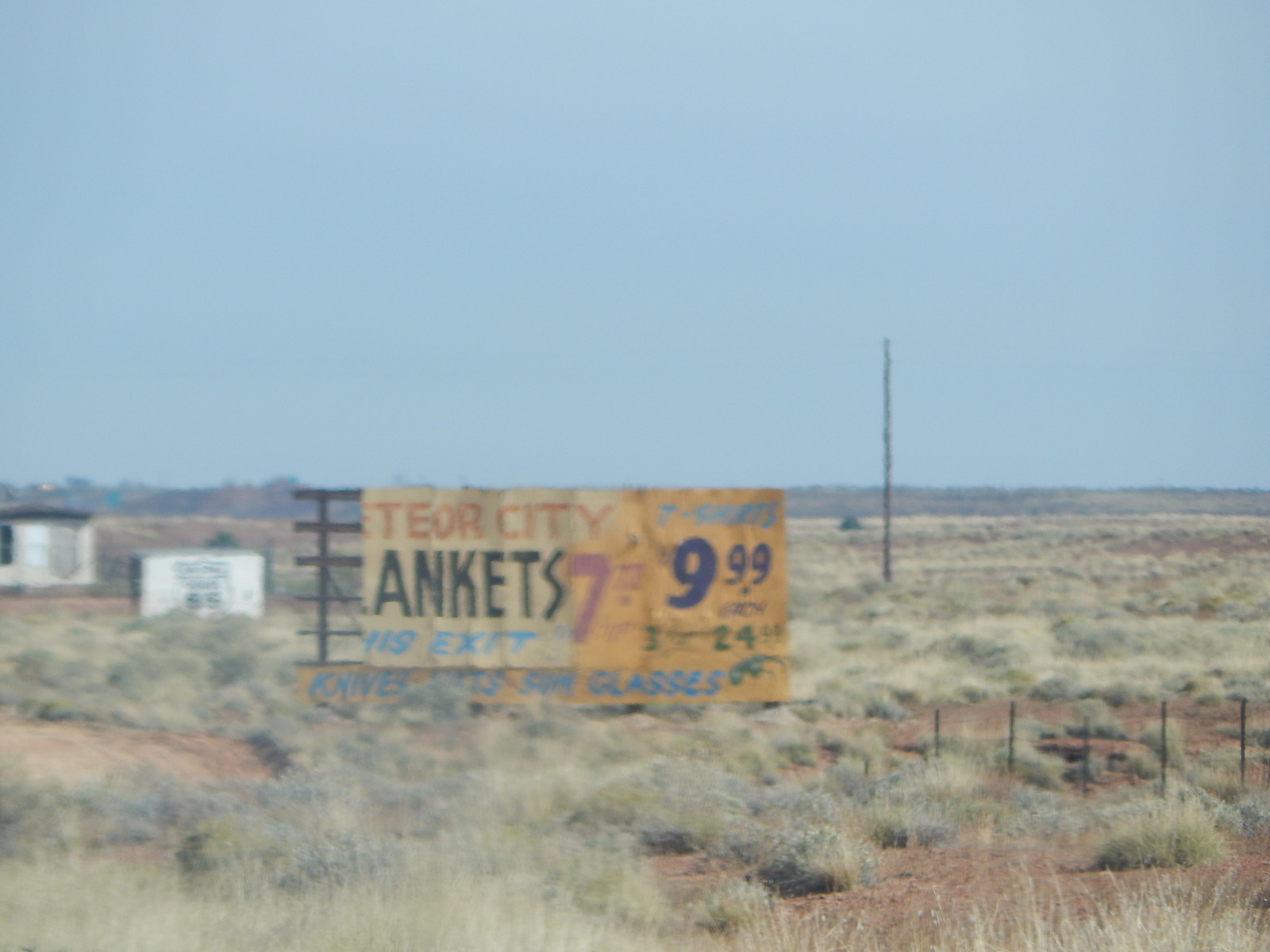The image presents a first-person perspective of a weathered sign positioned in a paddock by the side of a road. The sign sits on a downward slope from the viewer's vantage point, partially obscured by thick, uneven patches of grass and bushes that lack the lushness of greenery, appearing a whitish-tan color, likely dried out from exposure to the sun. The paddock is enclosed by a small, rustic cow fence, hinting at a rural setting.

The overcast sky above is tinged with a blue hue, indicating a mix of cloud cover and fog. The sign itself, displaying an older design, is mounted on a sturdy frame that appears to be made of either wood or steel. Despite sections of the sign being cut off, the visible text reads "Harm the lift," though this is likely incomplete. Further decipherable fragments include "In ke TS," possibly hinting at "blankets," followed by "for something city," with the partial words "e te o our city."

Two prices are listed at the bottom of the sign: $7.99 in pink and $9.99 in blue-purple, adding a splash of color to the otherwise muted scene.